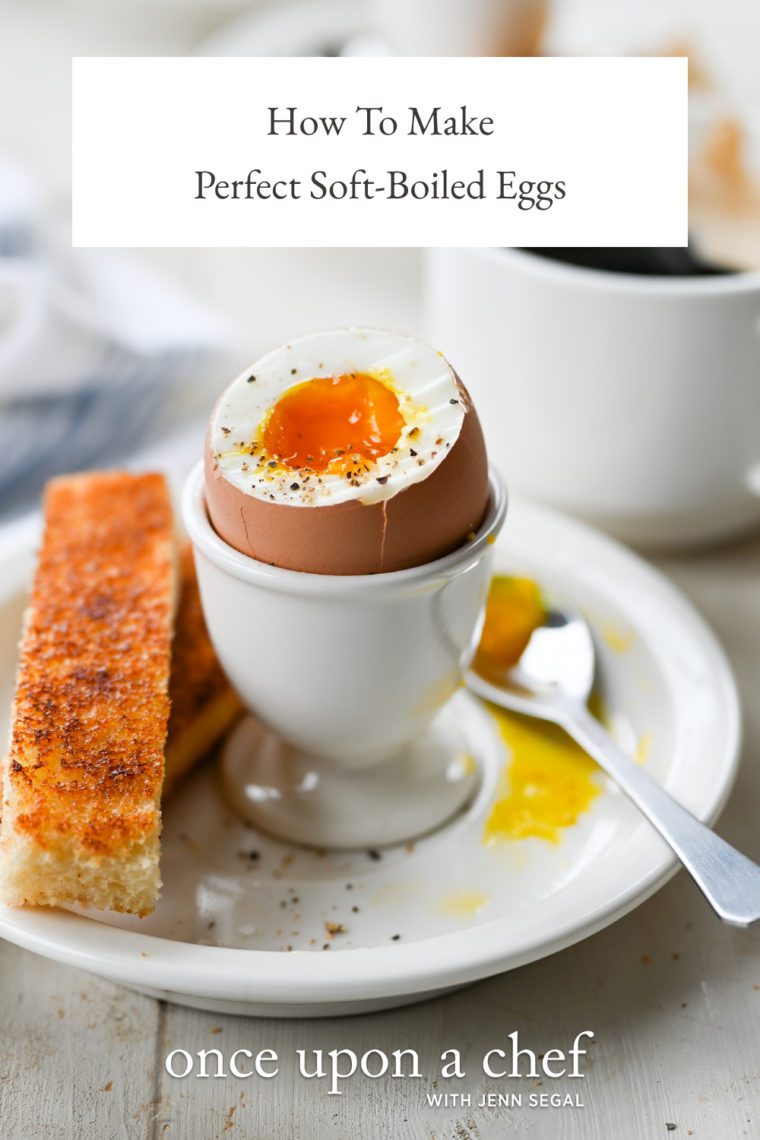The image is a highly detailed photograph that appears in a magazine or on a website titled "How to Make Perfect Soft-Boiled Eggs," prominently displayed in bold black text on a white rectangular bar at the top. At the bottom of the image, it reads "Once Upon a Chef with Jen Siegel" in white lettering. The central focus of the photograph is a soft-boiled egg, presented in a white ceramic egg holder. The egg has its top third removed, exposing its golden, runny yolk and the cooked white beneath. Surrounding the egg, placed on a shallow white dish, are several golden-brown breadsticks, ready for dipping. Additionally, a silver spoon rests on the dish, with a bit of egg yolk on its tip, suggesting it has already been used to sample the egg. To the top right of the image, there appears to be a cup of coffee, completing the inviting breakfast tableau.